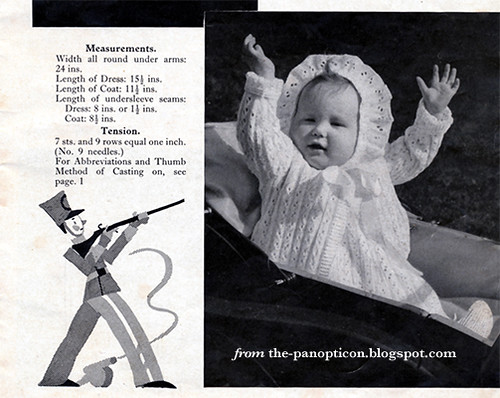This black and white image features a baby on the right side, dressed in a one-piece outfit with an attached bonnet adorned with eyelets. The baby is sitting in what appears to be a pram, with both arms raised beside its head. The baby’s outfit also includes a white sweater with a bow, and a matching gown. The background behind the baby is black.

Below the baby, a caption reads "from the dash panel piccon.blogspot.com." On the left side of the image, a white background contains various measurements in black text, including "width all around under arms: 24 inches," "length of dress: 15.5 inches," "length of coat: 11.5 inches," and "length of under sleeve seam: dress 8 inches or 1.5 inches, coat 8.5 inches." Additional details mention "tension: 7 stitches and 9 rows equal 1 inch, number 9 needles. For abbreviations and thumb method of casting on, see page 1.” At the bottom of this textual area, there is a cartoon illustration of a soldier shooting a gun.